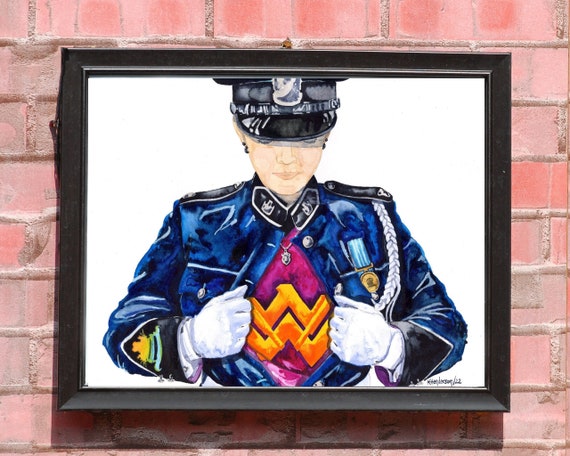The image features a salmon-colored brick wall with light beige mortar lines visible between the bricks. Centered on this wall is a black-framed photo with a white background. The photo captures an illustration of a woman dressed in a navy blue police or military ceremonial uniform, complete with shoulder lapels, a glossy-brimmed hat, and a looping white rope on her left shoulder. She is adorned with a medal, has white gloves, and is pulling open her jacket to reveal a magenta top with orange zigzags underneath, reminiscent of a Wonder Woman outfit. She appears to be wearing earrings, adding a subtle touch of femininity to her appearance.